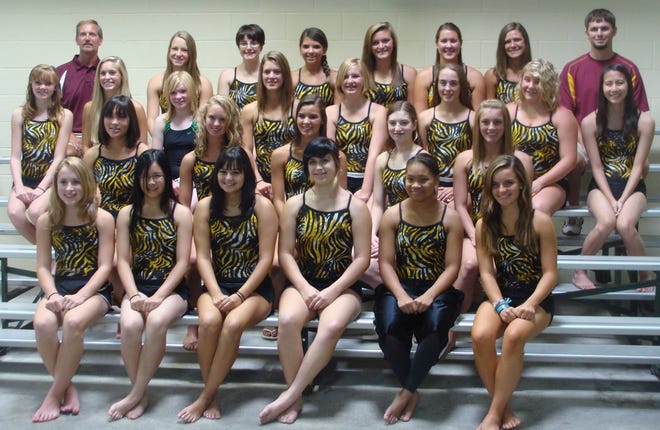The photograph features a group of girls sitting on silver metal bleachers inside a gymnasium, likely part of a sports team, possibly a swimming or basketball team. The girls are all dressed in swimsuits, characterized by a black background with yellow lines, and they are sitting in identical positions with their hands on their legs and their ankles crossed. One notable girl at the front left has light brown hair, while the next two girls over have long black hair, and the girl in the center sports short black hair. Another girl next to her, who has dark skin, is wearing pants and has her fists together at her knees. The girl next to her has dark brown hair parted to the left and is wearing a blue bracelet on one wrist. 

In the backdrop of the image, there are two men standing at the upper left and upper right corners of the bleachers. The man on the right is the tallest, has short brown hair, and wears an amber-colored shirt with a hint of yellow. The man on the left, who appears to be older with light hair and a mustache, also wears an amber shirt featuring a white strip.

Adding to the setting, behind the bleachers is a wall of white-painted cinder blocks, and the floor is concrete. None of the girls are wearing shoes, and many of them are smiling, contributing to an overall cheerful ambiance.